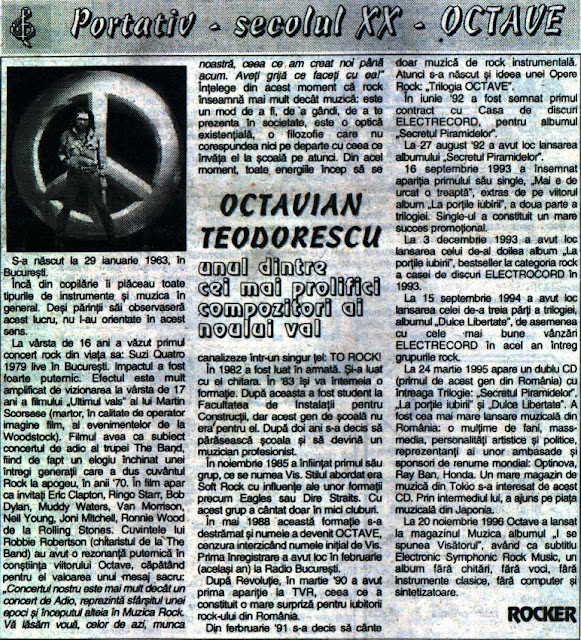The newspaper article, likely from the 1970s and in a foreign language, is headlined with "Portative Secolu XX Octave." At the top of the article, to the left, there's an image of a man with dark hair, dressed in a long-sleeved shirt and bell-bottom pants, standing with legs apart. This man is identified as Octavian Teodorescu, described as "uno d'entre semi-polifichi compositori ai Lului Ba." The upper left corner also features a large circle with a vertical line and two diagonal half-lines, resembling an upside-down peace symbol. The predominant colors of the image are black, white, and gray, with the lower right corner of the article prominently displaying the word "Rocker."